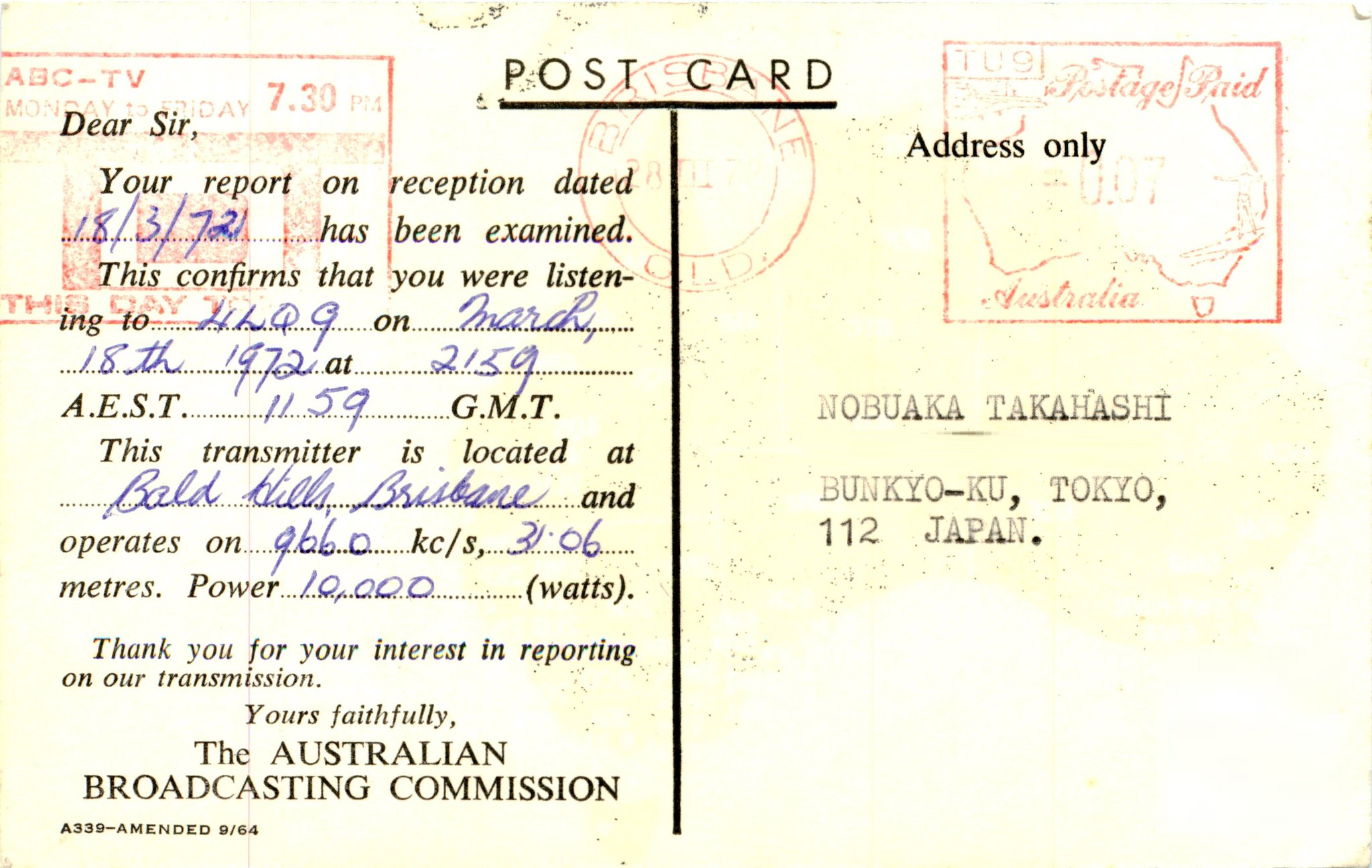This is an image of a vintage reception confirmation postcard from the Australian Broadcasting Commission. The postcard, which takes up the entirety of the image, prominently features a pink stamp in the upper right corner and is addressed to Nobuoka Takahashi in Bunkyo-ku, Tokyo 112, Japan, with typewriter print. The postcard's text, written in blue ballpoint pen, reads: 

"Dear Sir, your report on reception dated 18-3-72 has been examined. This confirms that you were listening to our station on March 18, 1972, at 21:59 AEST (11:59 GMT). The transmitter, located at Bald Hills, Brisbane, operates on 9660 kHz with a power of 10,000 watts. Thank you for your interest in reporting our transmission. Yours faithfully, the Australian Broadcasting Commission." 

The postcard is rendered in a palette of tan, red, pink, blue, grey, and white, reflecting its aged, historical nature.